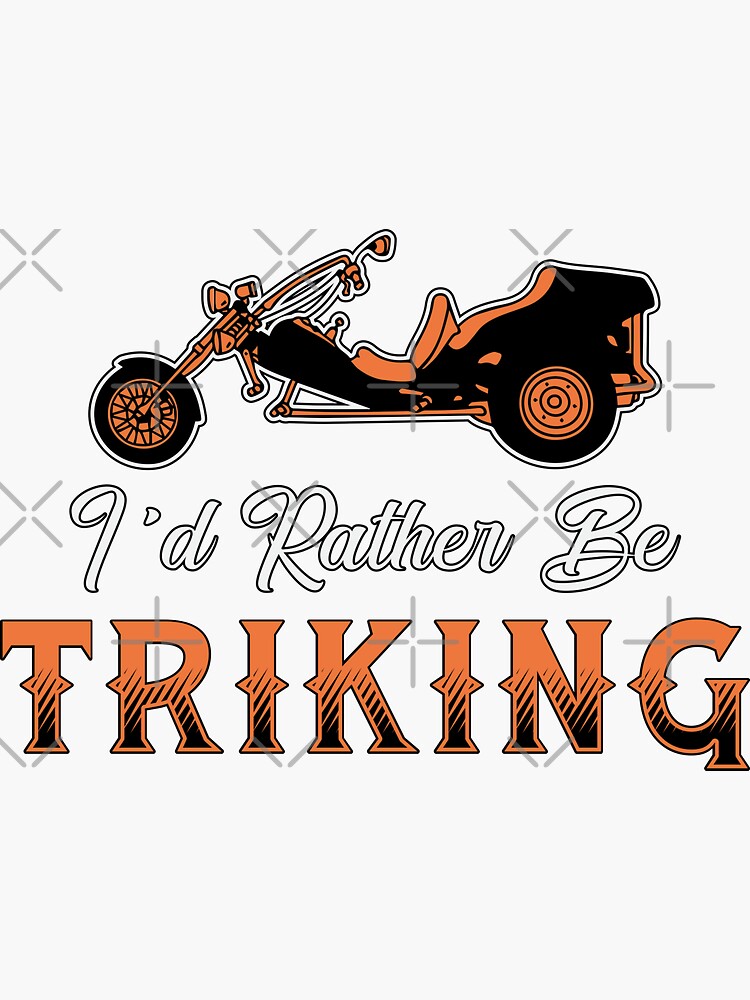The poster, primarily designed in white, black, and orange, features a repeating watermark of gray X's and pluses. The background of the poster is plain white. Central to the design is a prominent stylized illustration of a trike, resembling a motorcycle in a tricycle format, with a black body, orange highlights, black tires, and orange wheels. Above this illustration, large cursive white letters with black outlines spell out "I'd rather be," followed by the word "triking" in a bold, light orange block font shaded with hashed black lines at the bottom. The handlebars, headlights, and other trike details also incorporate the striking black and orange color scheme, creating a cohesive and visually engaging design.